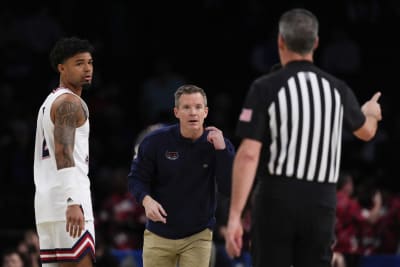The image portrays a tense moment during what appears to be a basketball game. On the left, there's a tattooed African American basketball player in a white jersey and white shorts with red, white, and blue stripes at the bottom. He is standing sideways, looking towards the center of the image. The middle figure is a middle-aged Caucasian man, likely a coach, with a graying, salt-and-pepper hair who is wearing a long-sleeved navy jacket and beige trousers. He has his mouth open as if speaking, and his left arm is raised in a gesture. To the right, facing both these figures with his back to the viewer, is the referee. He is wearing the quintessential black and white vertically striped shirt with black pants. The referee's right hand is extended, pointing to his right, indicating he might be addressing an issue. The background is predominantly dark, with a blurred section hinting at a crowd of spectators.